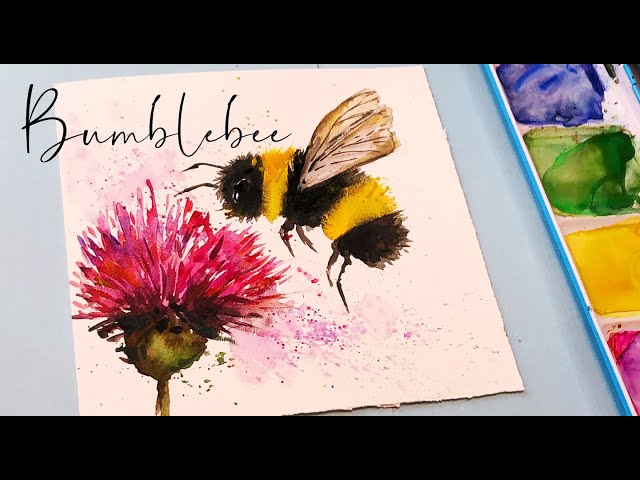The image is an indoor photograph of a painting, still likely in progress. The overall photograph is rectangular, about four to five inches wide and three to four inches high, with black borders about half an inch thick at the top and bottom. The primary background is light blue, and on the left side, there is a white piece of paper slightly tilted, with the right side higher than the left. 

The painting features a pink flower with thin, fine petals emerging from a light yellowish-brown and green stem, positioned in the lower left corner of the paper. Adjacent to the flower, a furry black and yellow bumblebee is flying towards it. The bee has a detailed structure with alternating black and yellow stripes, four legs, two feelers, and clear wings. Above the bee and flower, inscribed in black cursive writing on the white paper and extending slightly onto the blue background, is the word "bumblebee."

To the far right of the image, and partially overlapping the light blue background, a tray of watercolor paints is visible. The paints are arranged vertically with blue at the top, followed by green, yellow, and pink. The scene suggests an active painting environment, with attention to the tools and elements used in creating the artwork.